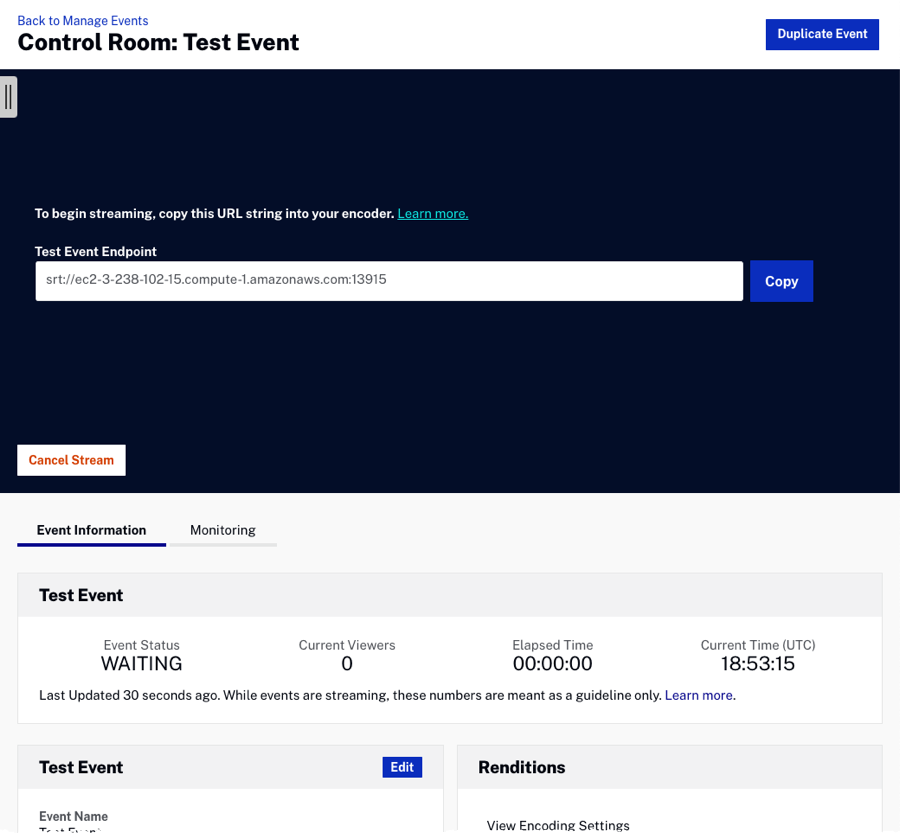The image is a screenshot of a web page titled "Control Room: Test Event." At the top, there's a blue rectangular button with white text labeled "Duplicate Event." The upper section of this web page is predominantly black, creating a clear contrast with the white elements. In the center of this section, a white rectangular input box is positioned below the instruction: "To begin streaming, copy this URL string into your encoder." Below this instruction, teal underlined text reads "Learn More."

Further down, the page displays "Test Event Endpoint" followed by a URL link within the white box, accompanied by a blue "Copy" button on the far right. At the bottom of this section, a white button bearing red text says "Cancel Stream." The lower portion of the image is segmented into two areas: "Event Information" and "Monitoring." Currently, the event status is displayed as "Waiting."